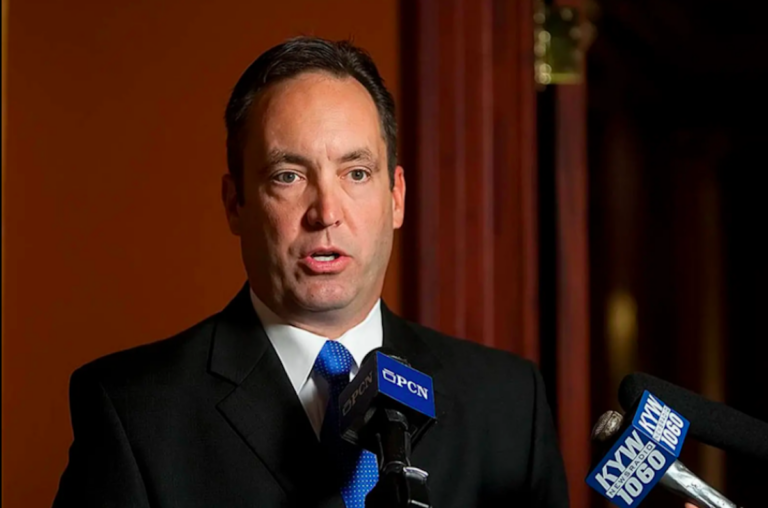This detailed photograph captures a middle-aged Caucasian man, estimated to be around 45 to 50 years old, engaging in what appears to be a serious discussion, possibly at a news conference. He is clean-shaven with very dark, short hair and has a light tan complexion. The man is seen from the chest up, wearing a black suit, a white shirt, and a distinguished blue tie adorned with small white dots. His mouth is slightly open as he speaks into a microphone. 

The main microphone in front of him sports a blue square label with white capital letters that read "PCN." Additionally, to the right of him, another microphone juts out, also featuring a blue square. This second microphone's label displays "KYW News Radio" and "1060" in white text. The background is predominantly a dark reddish-orange wall or curtain, with a portion on the right-hand side darker, possibly a dark brown or black wall, adding depth and contrast to the scene. The man's serious expression underscores the importance of the moment being captured.